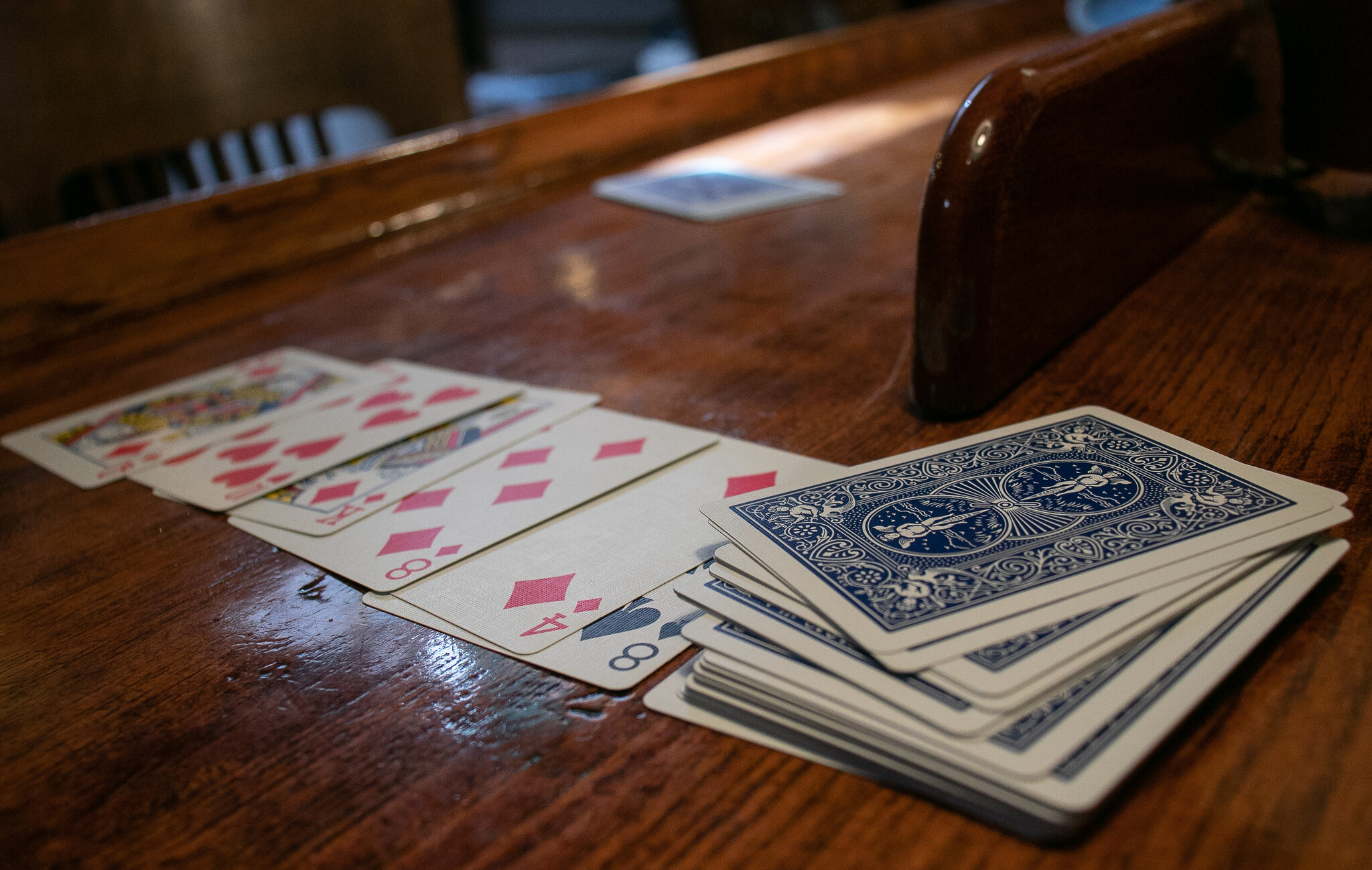A meticulously arranged setup features a stack of playing cards with blue backs, characteristically resembling traditional Bicycle brand cards, on a richly polished, dark-stained wooden desk. To the left of the stacked cards, six cards are spread out in the following order: the eight of spades, four of diamonds, eight of diamonds, king of diamonds, ten of hearts, and queen of diamonds. The desk itself is furnished with a protective wooden rail around its perimeter, matching the dark, polished finish of the desktop. Two chairs are partially visible in the scene; one is pushed under the desk from the upper left, and another is aligned to the upper center, suggesting the table's multi-purpose use. The overall composition exudes a sense of order and a touch of elegance, highlighted by the rich, dark wood and neatly displayed cards.